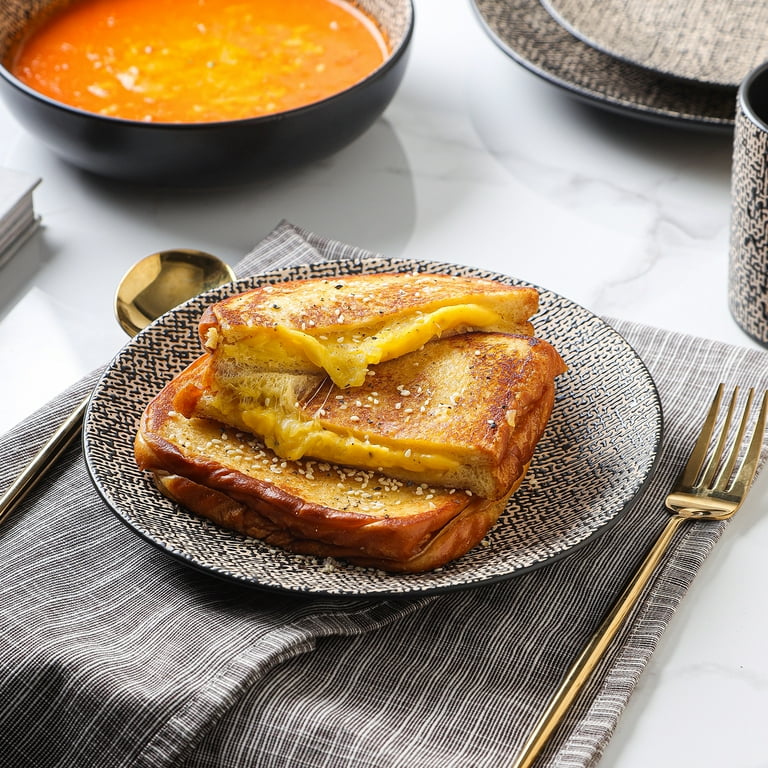This image depicts a cozy and inviting table setting for a solo lunch, featuring a classic pairing of grilled cheese sandwiches and tomato soup. The focal point is a blue and white plate, resting on a gray and white striped napkin. The plate holds three golden brown grilled cheese sandwiches, with cheese visibly oozing out from between the bread slices, some adorned with sesame seeds. To the right of the plate is a gold fork, and to the left, a gold spoon. Adjacent to the plate, there is a matching dark blue bowl filled with warm tomato bisque, topped with a sprinkling of cheese, which complements the sandwiches. In the upper right corner of the image, two stacked plates with a white crisscross pattern and blue edges are visible, accompanied by a matching blue mug. The setup suggests a serene solo dining experience, possibly accompanied by a book placed just slightly to the left of the main setting.